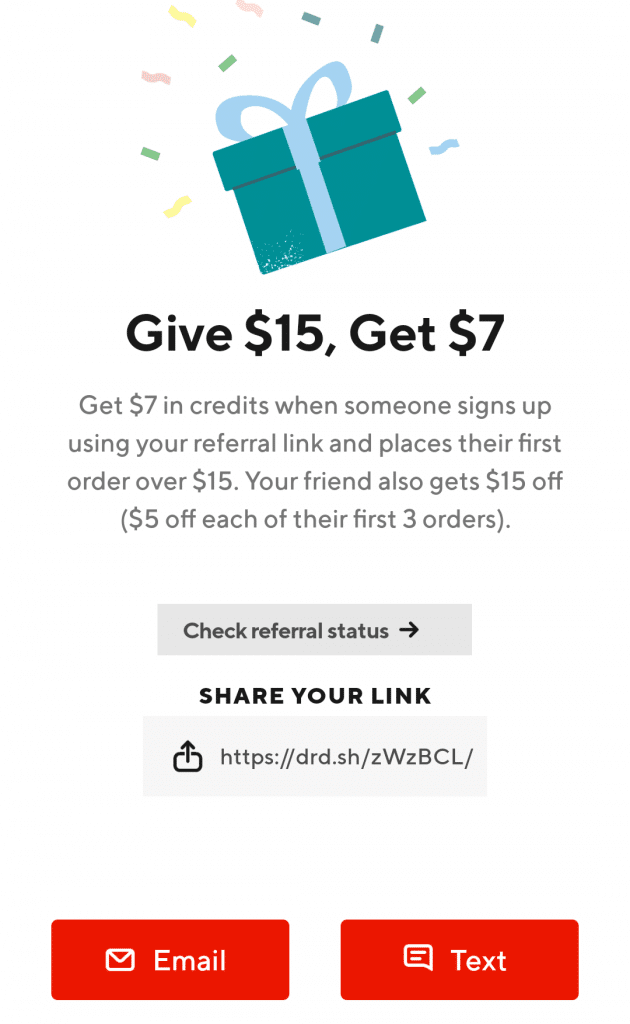Earn $7 in credits when someone signs up using your referral link and makes their first order over $15. Your friend also receives a total of $15 off, distributed as $5 off each of their first three orders. Check your referral status and share your link through this link: https://drd.sh.wzbcl/. The image features a blue gift box adorned with a lighter blue bow and ribbon, surrounded by floating confetti, creating a festive atmosphere.